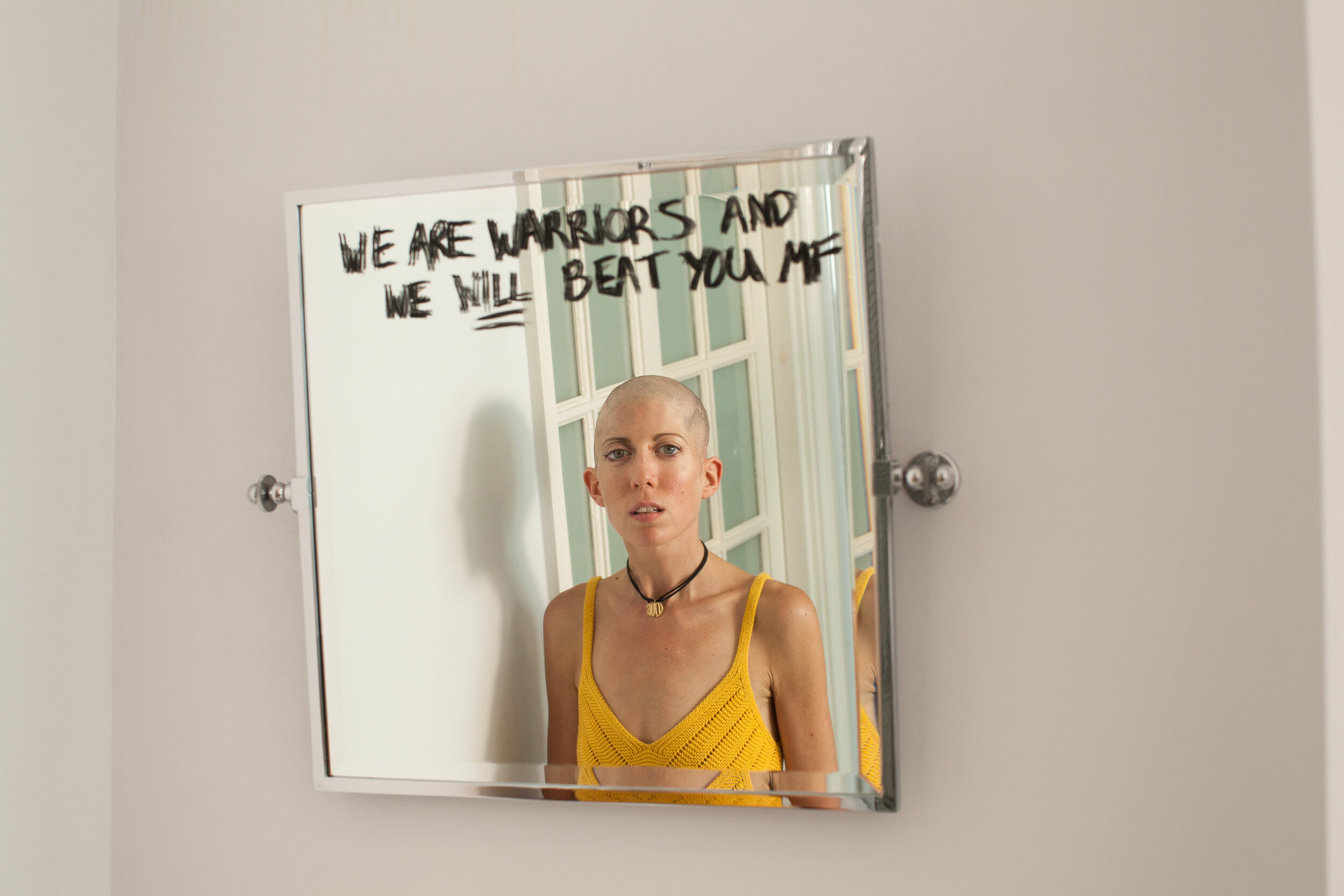In the image, a chrome-framed, square mirror is mounted on a uniformly painted wall — appearing white or tan — secured by brackets and visible screws at both sides. Reflected in the mirror is a bald woman with blue eyes, wearing a yellow knit tank top and a black choker adorned with a yellow medallion. She stands in front of a door, casting a shadow on the wall behind her. Her expression is neutral, and she gazes directly at the viewer through the mirror. Notably, scrawled in capital letters across the top of the mirror, possibly in grease pencil, are the words: "WE ARE WARRIORS AND WE WILL BEAT YOU MF," with the word "WILL" double underlined. The acronym "MF" likely stands for "motherfucker," adding a defiant tone.